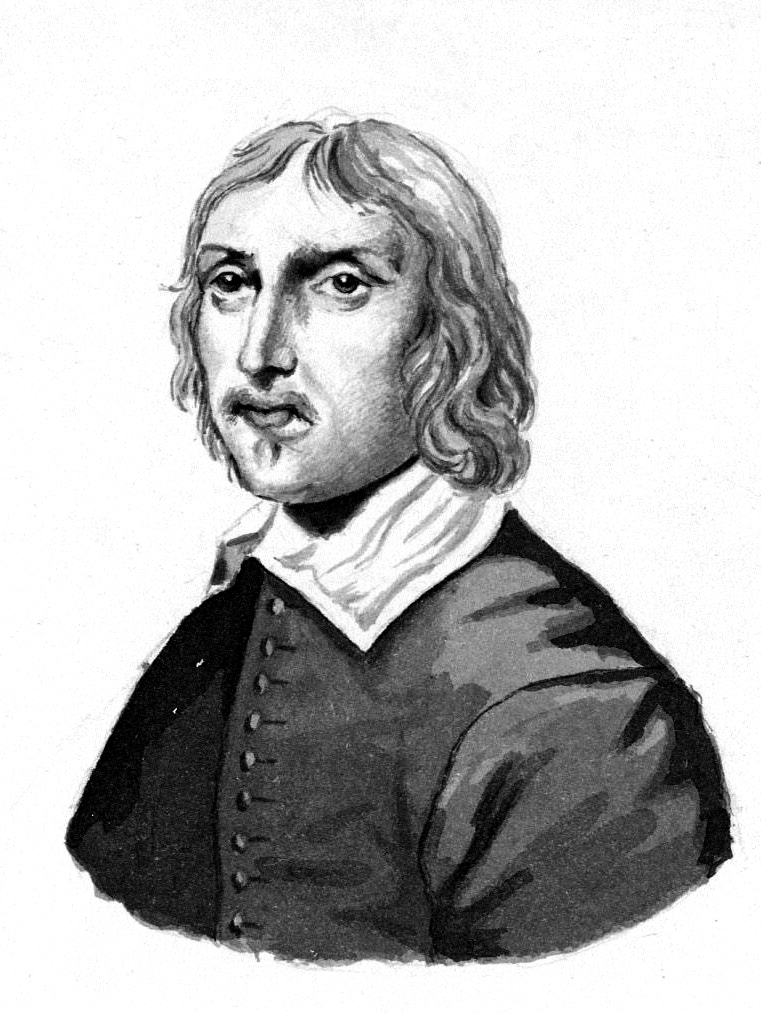This black and white illustration is a detailed portrait done in a watercolor style, capturing the likeness of a young man from a bygone era, possibly the 17th or 18th century. The man, seen from the chest up, sports medium-length hair that reaches near his shoulders. His face is characterized by wide features, a long, prominent nose, and eyes set somewhat far apart. A small mustache adorns either side of his upper lip, complemented by a modest patch of hair below his lower lip, resembling a goatee. His attire consists of a large, buttoned-up jacket layered over a white shirt with a prominent, thick collar. There is a solemn expression on his face, as he stares directly at the viewer, enhancing the traditional, historical feel reminiscent of old portraits often found in pamphlets from the 17th or 18th century. The monochromatic color palette of blacks, grays, and whites adds to the vintage tone of the piece.